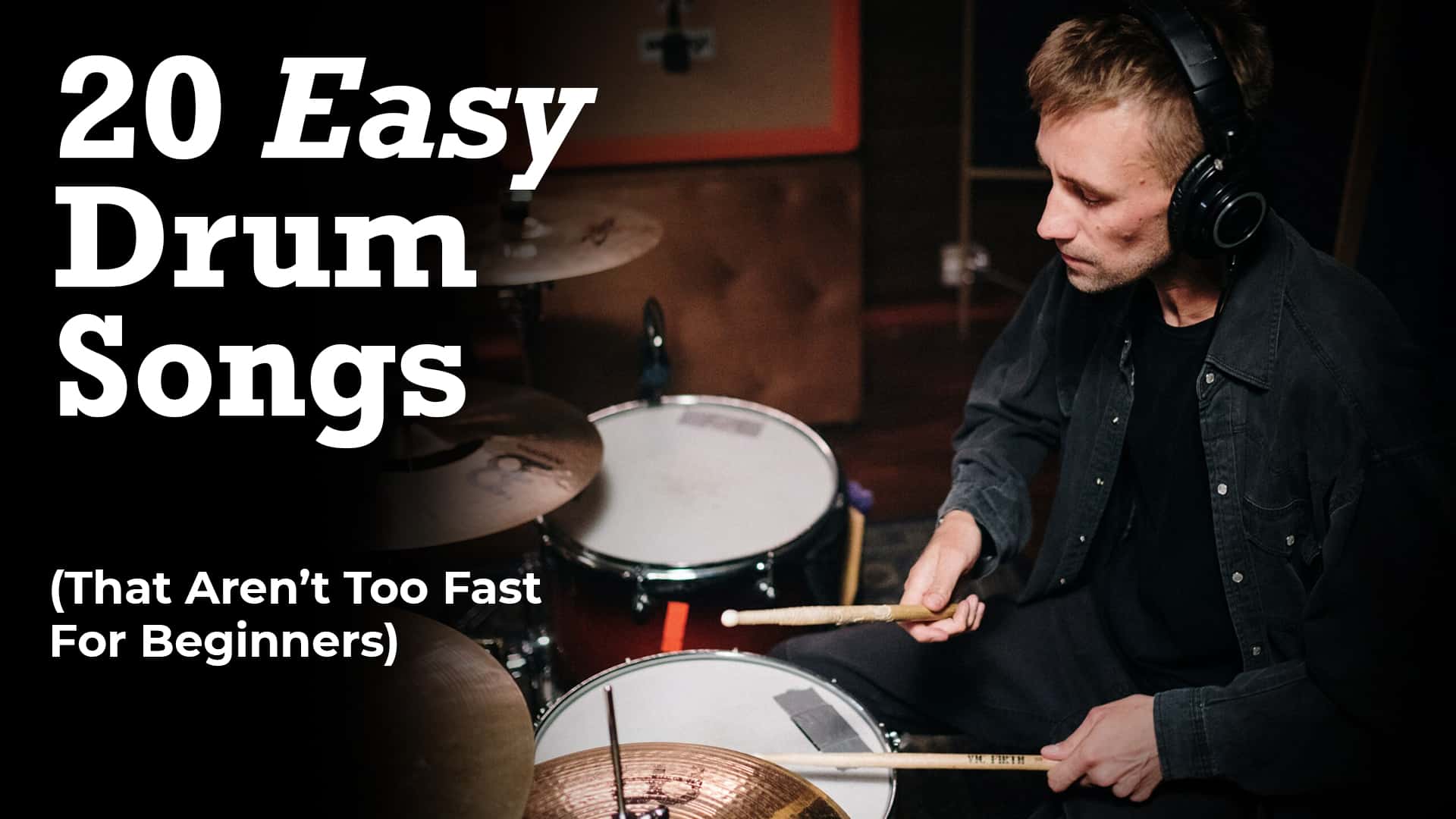In this color photograph, a man with blonde hair is depicted in a seated position playing the drums. He is centered towards the right side of the landscape-oriented image, facing left, and viewed from the top of his head down to his mid-hip. The man is wearing black headphones with silver accents, a black overshirt, black undershirt, and black pants. He is holding brown drumsticks over a white drumhead, with an orange and black patterned drum body.

The background comprises several layers: a tan carpeted wall, a brown brick wall, and a brown-framed window positioned behind the man's head. Beneath the drum set, the floor transitions from brown wood to a blue, gray, and white patterned carpet. A white wall switch and a black microphone with an orange detail are also visible in the background.

On the left side of the image, bold white text reads "20 easy drum songs," with a parenthetical note below, "that aren't too fast for beginners." The photograph captures the realism of the scene, combined with a graphic design element due to the text overlay, suggesting it might be a book cover or a website image.